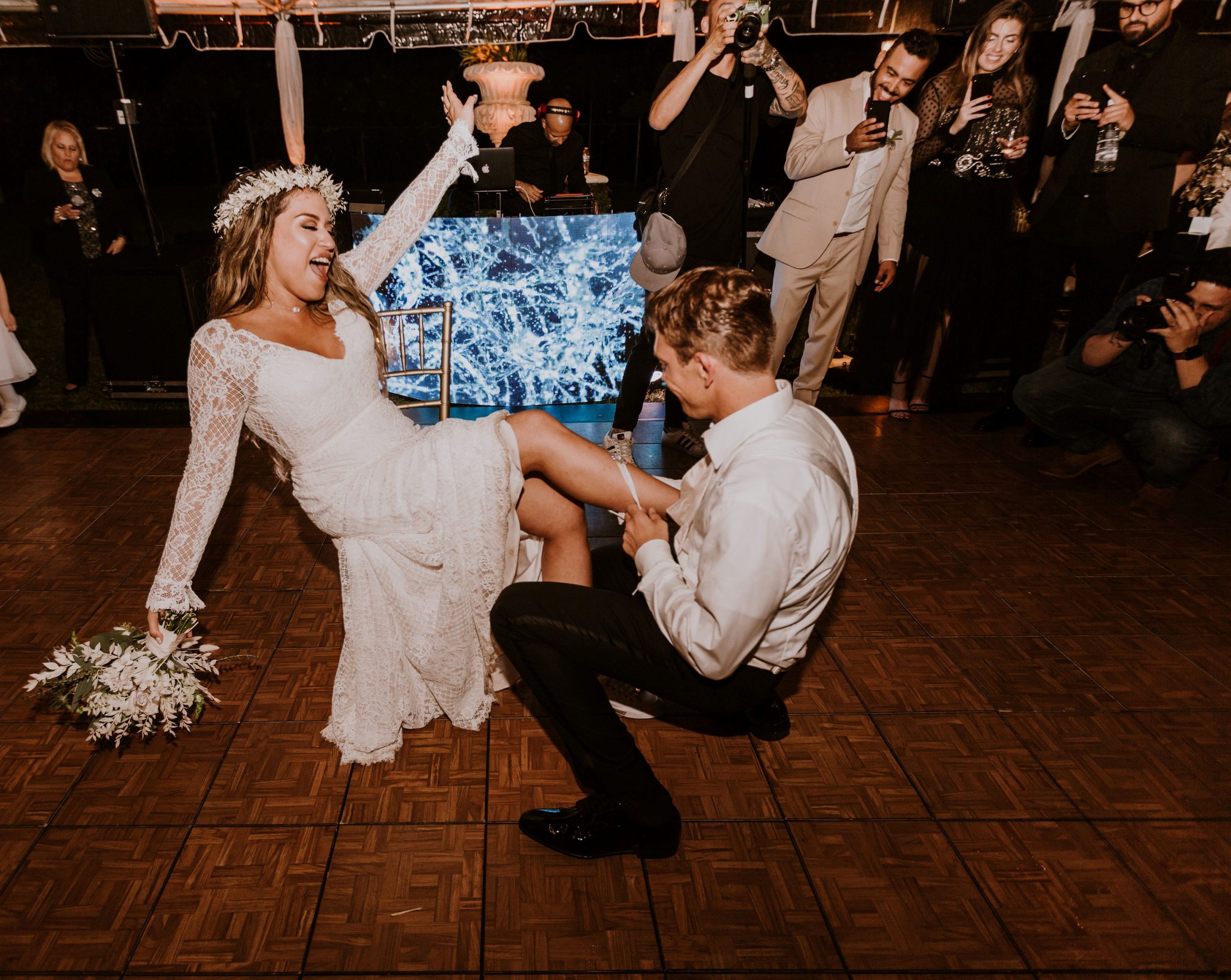In this vibrant image of a wedding reception, the joyful focus is on the bride and groom during the lively garter removal tradition. The groom, a young man with brown hair, is dressed sharply in a white shirt, black dress pants, and black dress shoes, captured from a side view as he squats to remove the garter from the bride's leg. The bride, stunning in her white wedding gown and a delicate white flower crown, leans back on a chair with a bright smile, her right hand holding a small dangling bouquet of white flowers. Her left arm is raised, adding a joyous flair to the moment. The setting is a wood dance floor with a dark brown rectangular pattern, surrounded by guests who are eagerly filming the event with their phones. Also present are two professional photographers meticulously capturing the scene. Behind the couple, the DJ is at his booth, which is lit with vibrant blue LED lights, creating an electrifying backdrop that accentuates the festive atmosphere of the reception. A woman on the back left is seen looking at her phone, adding to the modern touch of the celebration. This detailed image encapsulates the exuberance and communal joy of the wedding celebration.